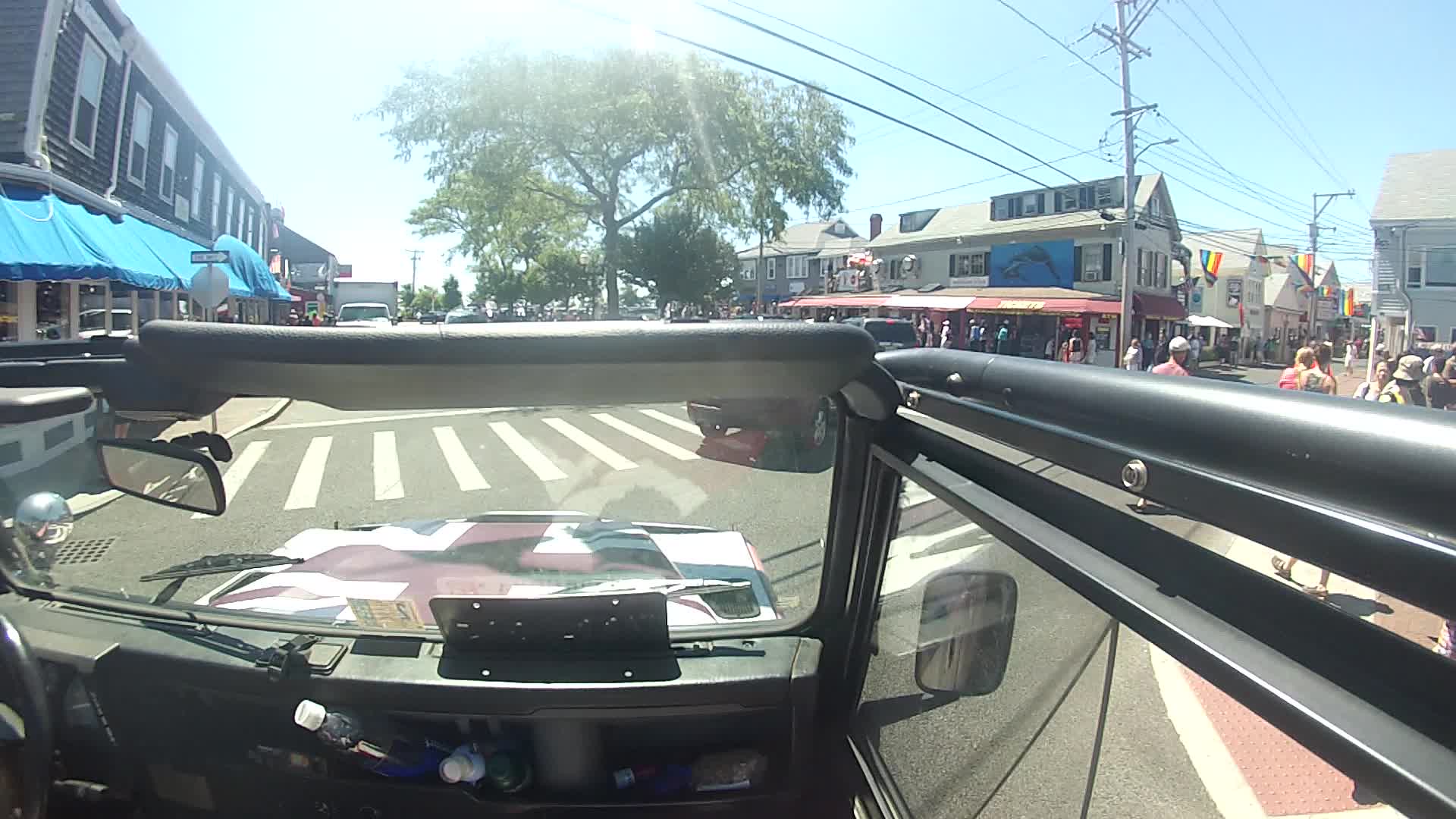The photograph, taken from within a roofless jeep-like vehicle, captures the vibrant scene of a small town, possibly during a pride parade. The image showcases the dashboard and front glass windows of the jeep, suggesting the photographer might be standing and leaning out where a roof would be to take the shot. The street veers off to the right, adorned with numerous rainbow flags, indicative of the celebration. The left side also features a similar setup of various vehicles and buildings. The town is bustling with pedestrians, highlighted under a clear blue sky suggesting midday. Trees with dense foliage can be seen, casting shadows and contributing to the warm and sunny atmosphere. The scene includes a mix of residential homes and small businesses, all framed by power lines overhead. Beams of sunlight filter through the trees, creating a hazy, picturesque effect, enhancing the overall charm and lively spirit of the photograph.